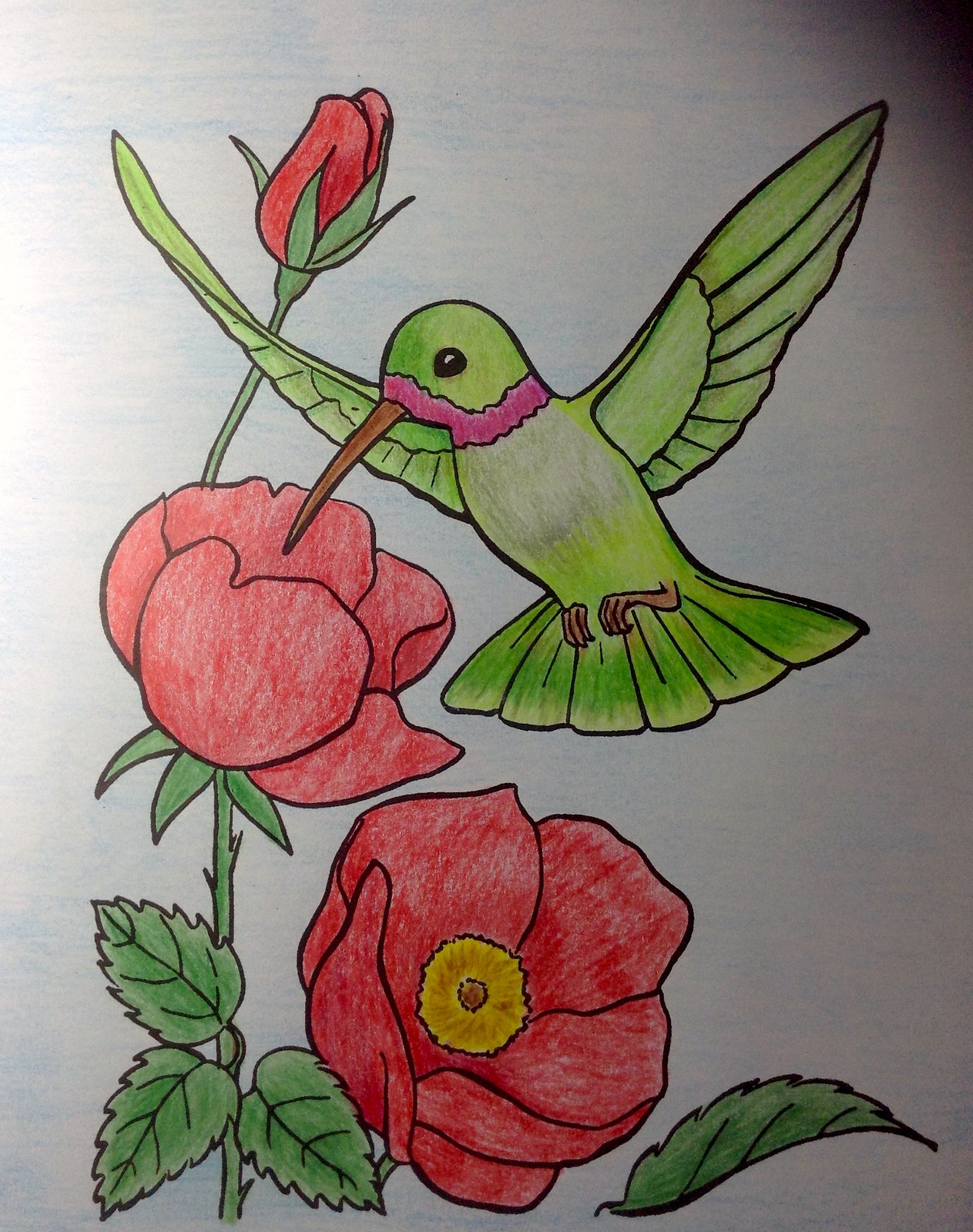This is an artistic drawing created on white paper, reminiscent of a coloring book page due to its black outlines. The illustration appears to be colored in with crayons, contributing to its charming, handcrafted look. The focal point consists of two vibrant red flowers with bright yellow centers located on the left side of the paper, each supported by a prominent green stem. Higher up, a red flower bud is depicted, not yet in bloom. In the upper half of the drawing, a green hummingbird is portrayed in mid-flight with its long brown beak poised to sip nectar from one of the red flowers. The hummingbird features a distinctive pink marking that extends down the front of its face and around its neck, adding a touch of vivid detail to the scene.